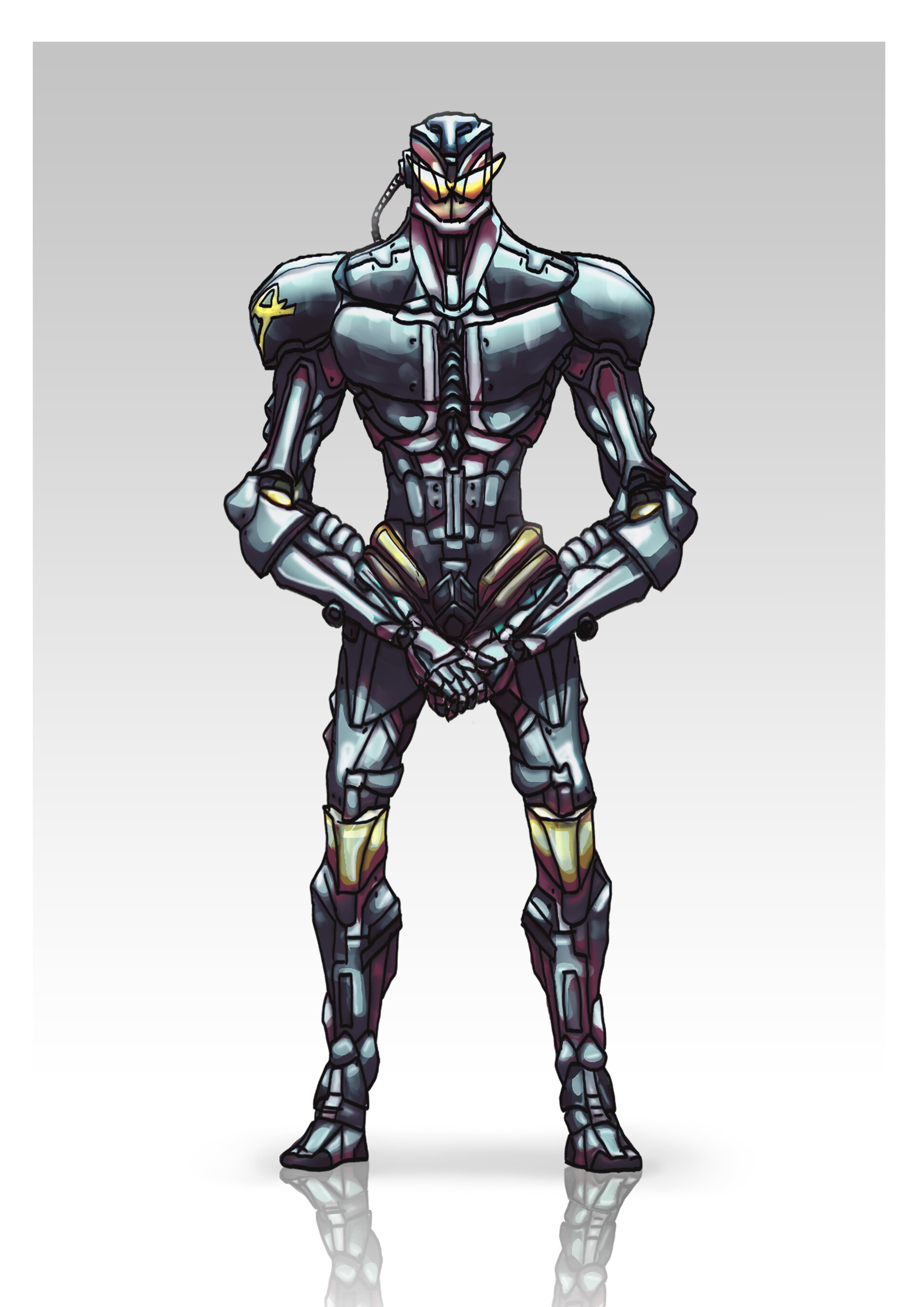The image depicts a comic book-style character resembling a superhero or sci-fi cyborg. The character, placed against a gradient background transitioning from purplish at the top to faint white at the bottom, is depicted standing with a reflective shadow beneath. The character appears to be constructed from various materials, predominantly metal, with a striking combination of colors. The head is adorned with a silver and red headpiece, accompanied by gold reflective shades. Its small head proportions suggest a non-human origin, reinforced by the presence of a conduit running from its ear to its back.

The torso, arms, and legs are primarily dark gray metal, exhibiting occasional blue hues. The knees stand out with shiny yellow and red tones, while the red and black calf sections lead to gray metallic shins and feet. A notable detail includes a yellow mark on the character's left shoulder. The figure evokes the aesthetic of iconic figures like Iron Man but stands apart with its unique blend of features and color scheme, lending it an air of a futuristic, armored hero or cyborg.